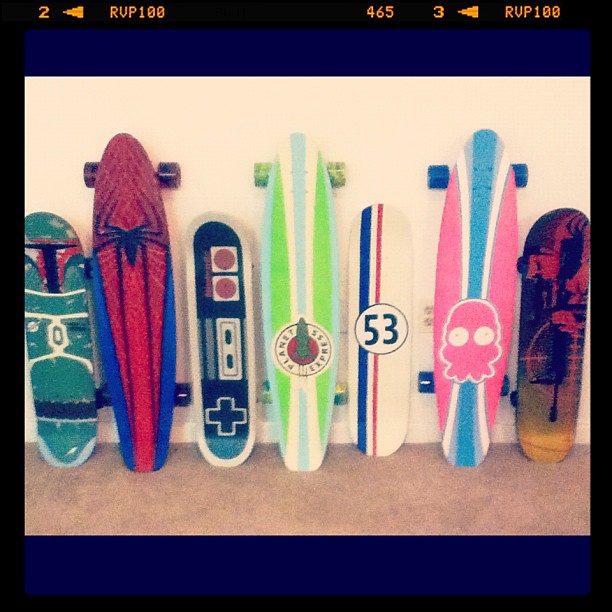The image features an array of seven skateboards and longboards, each adorned with distinct and vibrant designs, laid out on a beige rug. In the sequence from left to right, the boards exhibit the following designs: the first board showcases a Star Wars character, potentially the Mandalorian in his iconic green suit and helmet; next is a longboard with a Spider-Man theme, featuring a hybrid spider-suit design; following that is a skateboard with a retro Nintendo controller graphic. The fourth board displays the Planet Express logo from Futurama, with a green, white, and blue color scheme. Next is a skateboard marked with the number 53, encircled by striped red, white, and blue accents, reminiscent of Speed Racer or Herbie. The penultimate board is a longboard with a pink, blue, and white color palette, featuring a distinctive skull or octopus-like motif. Finally, the rightmost skateboard has an intense image of a figure, fully attired in red and brandishing a gun, with a yellowish gradient at the bottom.

The image appears to be a screenshot with various on-screen details: in the top left corner, there is a '2', a left-pointing triangle, and the letters 'RVP100'. The top center of the image shows the number '465', while the top right mirrors the left corner with the number '3', another left-pointing triangle, and the letters 'RVP100'. The composition is framed by a blue border along its edges, encapsulating this vivid display of skateboard artistry.